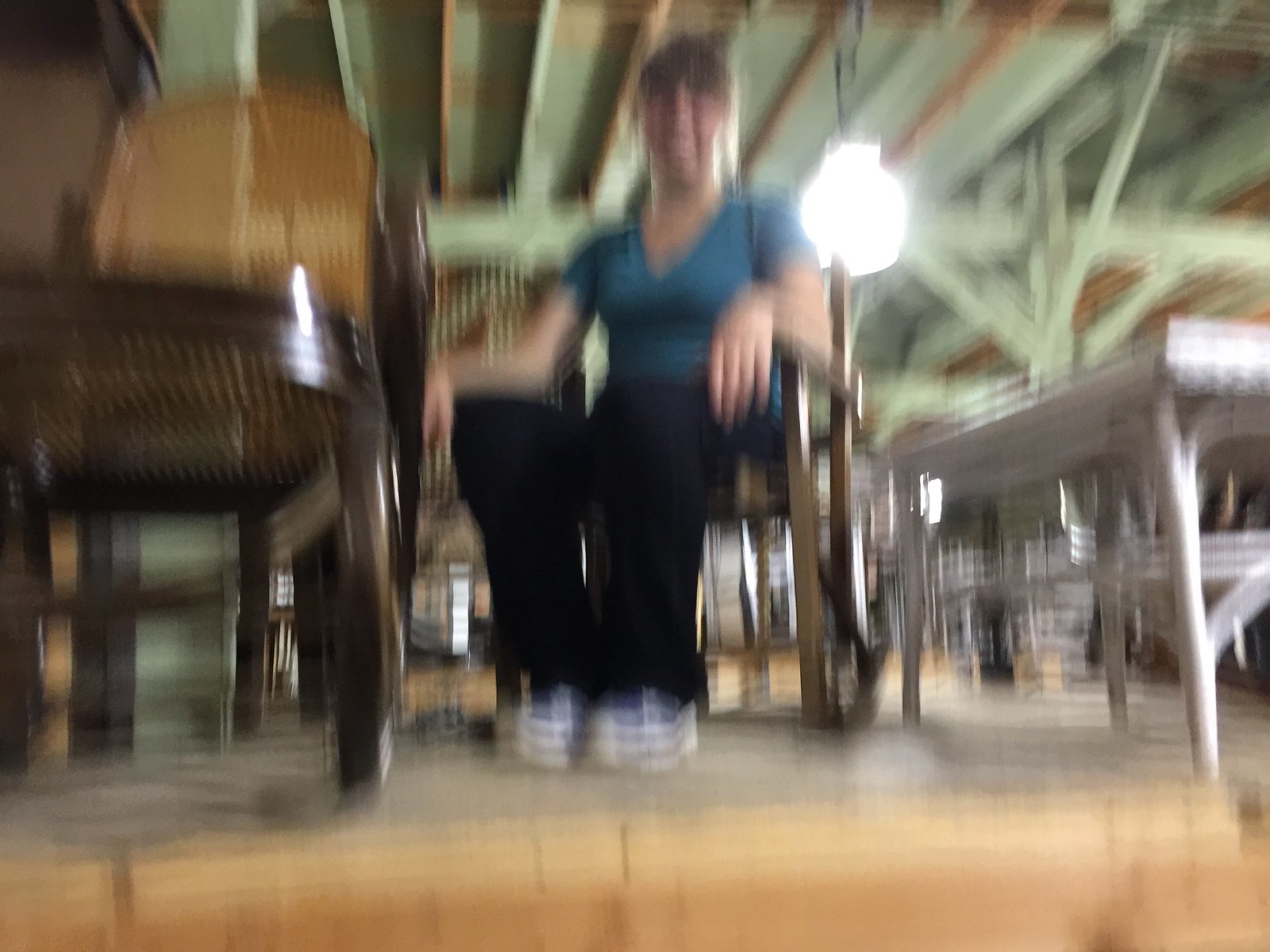The photograph captures a woman seated in a chair amidst a very blurry and shaky setting. The image quality is so poor that it's almost painful to look at, with the scene obscured by a bright glare possibly from an overhead light. The woman, who has a lighter skin tone and dark hair pulled back, appears to be smiling. She is dressed in a short-sleeved, sky blue v-neck t-shirt, paired with black trousers, and white and blue sneakers. She sits on a dark brown wooden chair with a lighter brown backing. To her right, there's another chair, which is dark brown with a light brown woven backing. A white coffee table can be seen on her left. The room has a tan white wooden floor and green wooden ceiling with boards. There’s a white bench or tabletop on the right and another table on the left. Overall, the scene behind her is bright and contributes significantly to the image's blurriness.